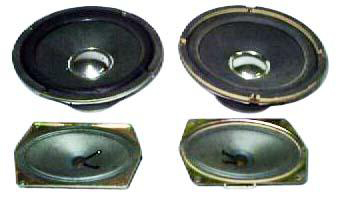The image features a pair of black subwoofers with distinct rings around them—one with a yellow ring on the right and the other with a black ring on the left—set against a white background. Both subwoofers have a silver circular part in their centers. Below these subwoofers are two smaller, curved silver components with black wires emerging from their centers. The overall picture is very small, with each component measuring about an inch, and it appears blurry, likely captured with an old digital camera or early cell phone. The subwoofers and the smaller components, possibly treble speakers, seem to be part of a disassembled speaker system laid out flat, providing a detailed yet nostalgic glimpse into older audio technology.